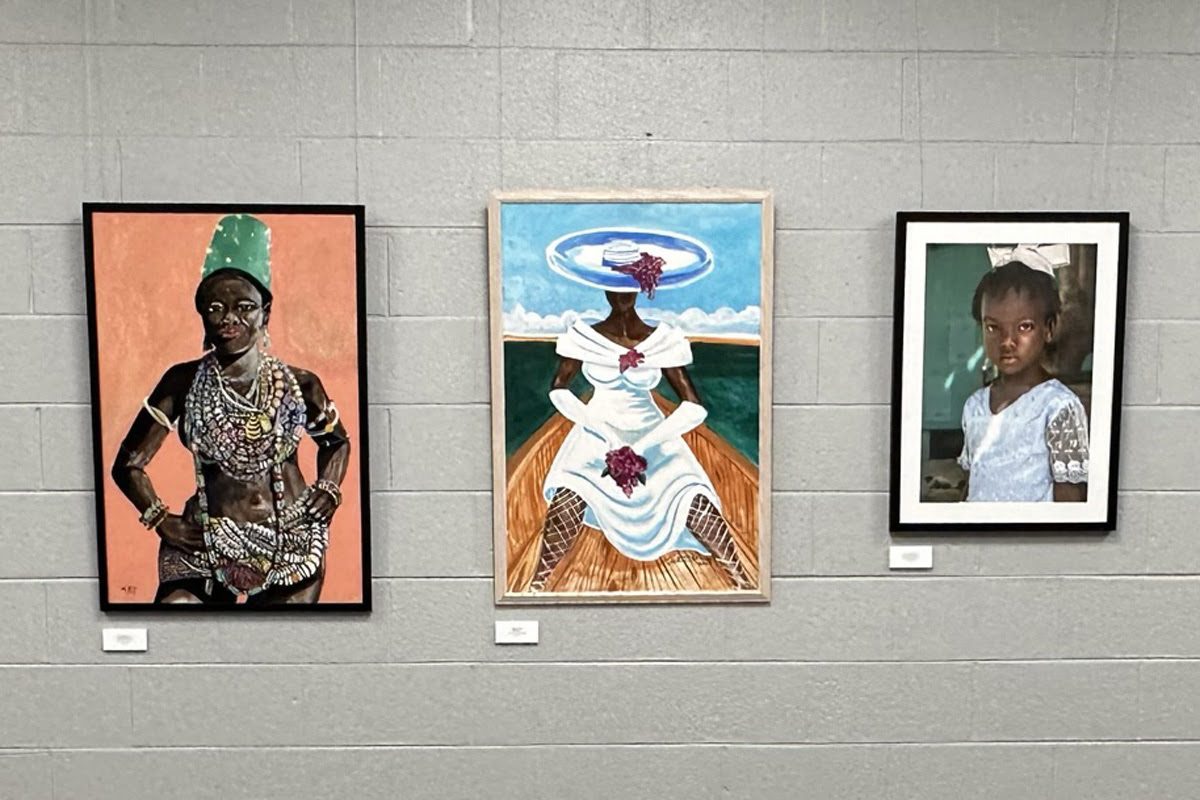The image portrays three framed artworks displayed on a textured gray brick wall, arranged in a slightly ascending order from left to right. The first artwork features a black woman adorned in traditional indigenous attire, with elaborate beads draped around her body and a striking green hat with white spots. She stands against an orange background, and a small tag is visible beneath the frame. The middle piece depicts another black woman, elegantly seated in a brown boat, dressed in a white gown with a shawl collar and a wide-brim sun hat with a blue rim. She is holding a bouquet, and her legs are clad in fishnet stockings. The serene scene around her includes a light blue sky with clouds in the distance and green water below her. The final artwork is a photograph or a photorealistic image of a young black girl wearing a white lace-sleeved dress, facing the camera with a calm expression. She stands against a green background with sunlight filtering in. Each piece is meticulously framed and has a name tag beneath it, adding to the gallery-like presentation on the neutral gray wall.